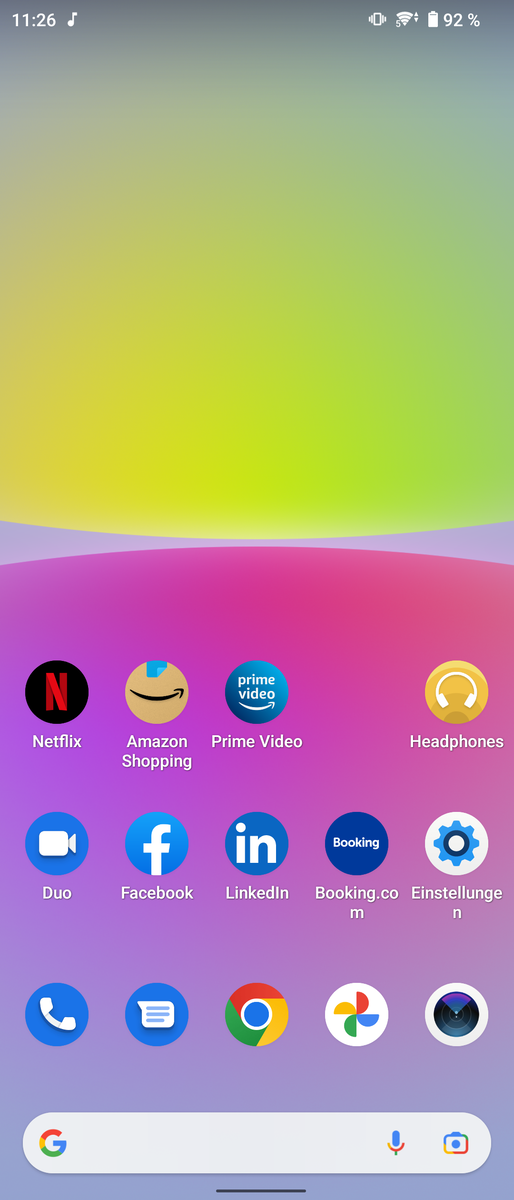The homepage of the cell phone features a simple, yet aesthetically pleasing background with an intricate ombre design. The top half of the screen transitions from a grayish color to an orangish hue on the left side, and from grayish to greenish on the right side. This gradient effect is mirrored horizontally, blending from a goldish shade to a greenish hue across the screen. In the middle, a subtle concave and convex sliver of light purple provides a distinct separation. Below this, another gradient pattern inversely replicates the top, transitioning from purplish to gray.

The middle section of the screen showcases a series of app icons neatly arranged. These include Netflix, Amazon Shopping, Prime Video, Headphones, Duo (a video app), Facebook, LinkedIn, Booking.com, Einstein Lunch, and Einstein Still Lunch. Essential utilities such as Phone, Text, and Chrome are also present. At the bottom of the screen, a Google search box is conveniently located for easy access.